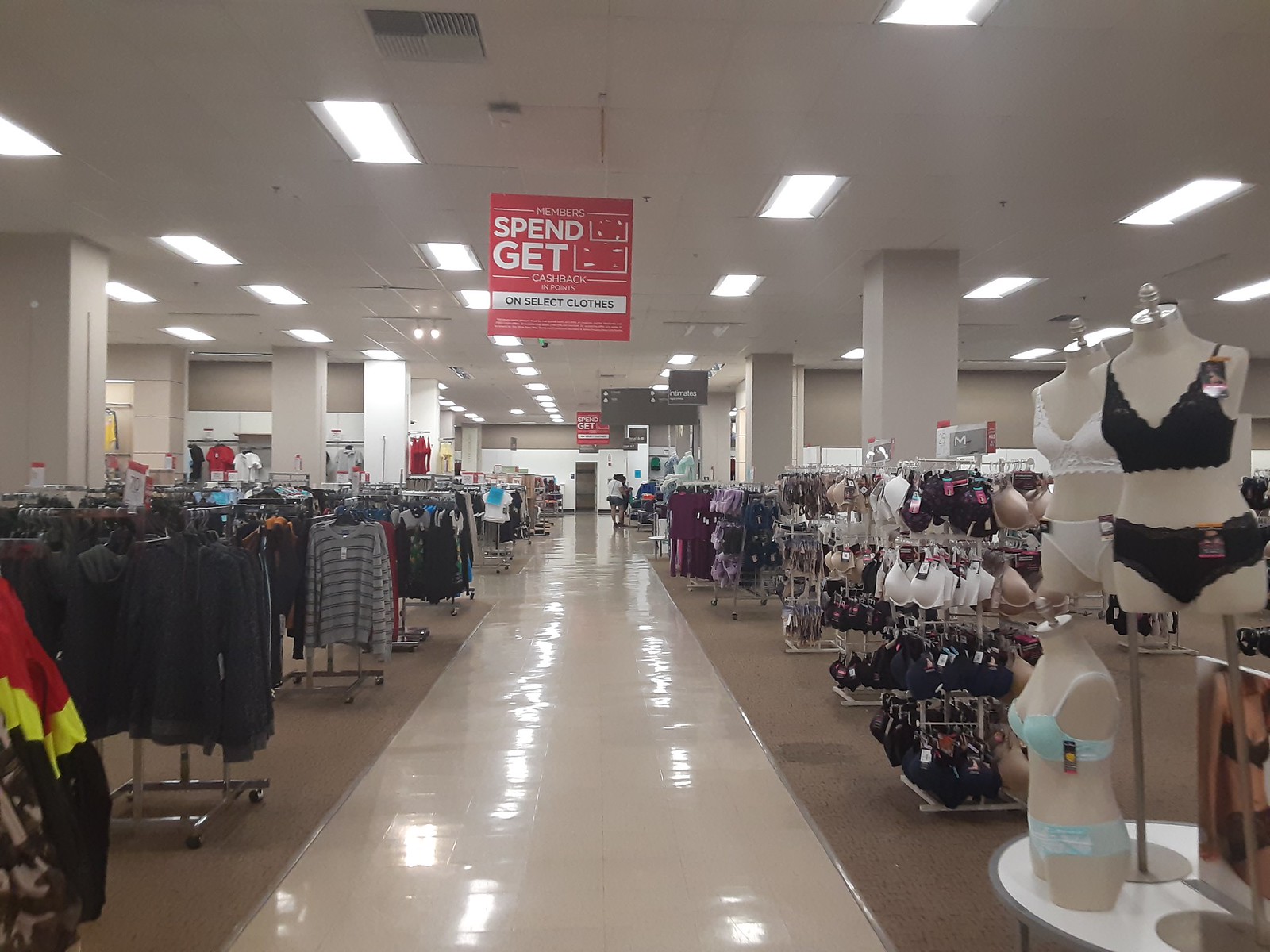The image depicts the interior of a brightly lit department store, featuring a wide aisle with white or light tan tile flooring flanked by beige or brownish carpet on either side, designating areas where the merchandise is displayed. The ceiling is a standard drop ceiling with evenly spaced rectangular fluorescent lights. On the right side of the aisle, there are displays of women's underwear, including bras and underwear showcased on mannequins. The left side of the aisle features men's casual clothing, predominantly dark sweaters, hoodies, jackets, and shirts, with t-shirts or short-sleeve polos visible further toward the back. A large red sign hangs from the ceiling, promoting a “spend and get cash back” offer on select clothes. The store appears to be spacious, extending far back where a couple of indistinct figures can be seen.